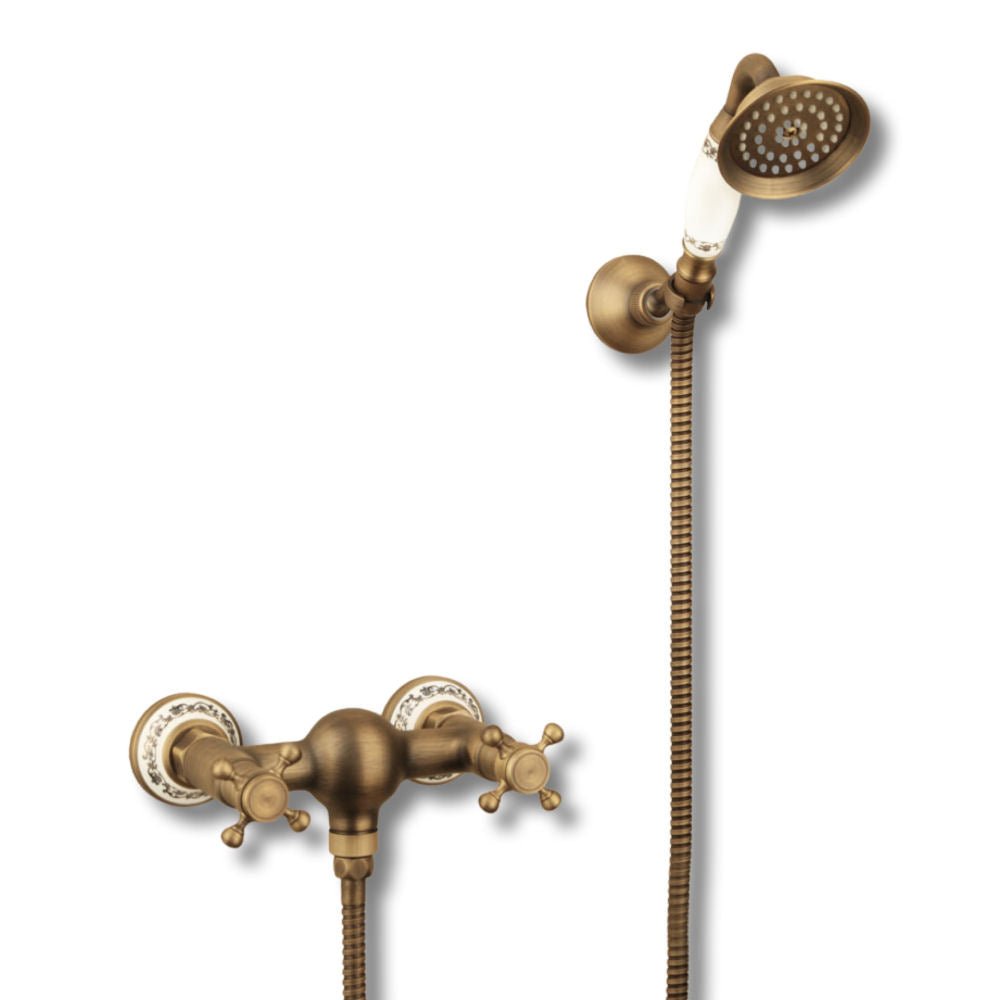The image depicts a luxurious, stock-photo-style setup featuring a sleek, brushed gold faucet and shower head against a pristine white background. Both the faucet and the shower head are made of a shiny gold or bronze material, with intricate detailing and elegant engravings. The faucet is wall-mounted, secured by two circular white porcelain fixtures with gold scrollwork. It includes two spigots for hot and cold water, positioned on either side of the central, decorative gold sphere. From this sphere, a spiral, rod-like connector extends, also in gold, linking the faucet to the handheld shower head. The shower head possesses multiple tiny holes for the water to spray through and features a handle crafted from white porcelain, edged with gold etching that matches the attached fixtures. The overall design merges functionality with opulence, showcasing a harmonious blend of white porcelain and luxurious gold elements.